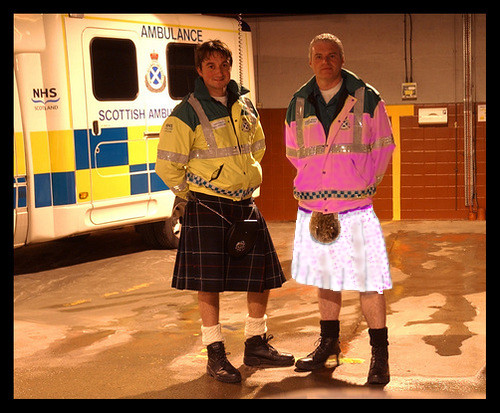The photograph captures a candid moment of two men standing outdoors, centered in front of a white Scottish ambulance with blue and yellow checkering. The ambulance bears the text: "Ambulance," "Scottish Ambulance," and "NHS." The men are positioned against a background featuring a wall comprising two shades of brown tile and brick. The ground beneath them is a grayish-brown. 

On the left, a young man with dark hair dons a yellow, reflective emergency responder jacket paired with a dark-colored kilt and dark shoes. Beside him, an older man with short, bleached blonde hair wears a hot pink, reflective jacket. His attire includes a white kilt with a pink print, black socks, and black shoes, which appear to have heels. The scene, seemingly captured at night due to the lighting, is informal and likely taken by a bystander. The various elements of color include white, yellow, blue (from the ambulance), alongside the peach, gray, brown, green, yellow, black, and touches of gold from the men's clothing.